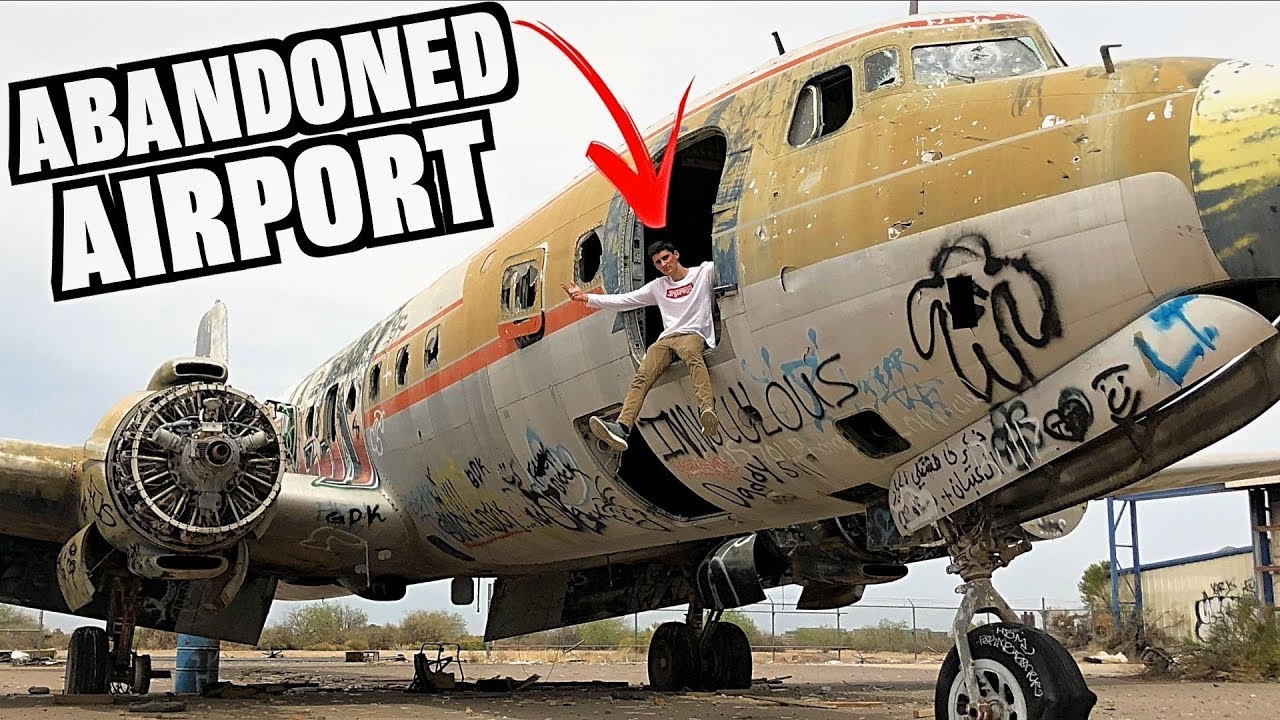This image depicts an old, abandoned passenger airplane situated in what seems to be a neglected airfield or storage area. The plane, once capable of holding approximately 30 passengers, is now in a state of disrepair, covered in various graffiti and with pieces of its metal housing pulled away. The top half of the plane is painted in a tan color with an orange stripe along the middle side, while the underside is white. The aircraft's windows are shattered, its wheels (with some illegible white markings) are intact but flat, and the engine cover is missing, exposing the blades.

Perched casually at the doorway—where the plane door should be—is a teenage boy with dark hair. He is dressed in a long white shirt, tan pants, and gray sneakers. His legs dangle from the opening, and he has one hand extended outward. Behind the plane, a small building and some fenced-in areas are visible. The setting is accentuated by clear skies and greenery from surrounding trees and bushes. In the top-left corner of the image, a label in white, all-caps lettering outlined in black reads, "ABANDONED AIRPORT." Notably, a red arrow points to the young man, emphasizing his presence in this scene of bygone aviation.